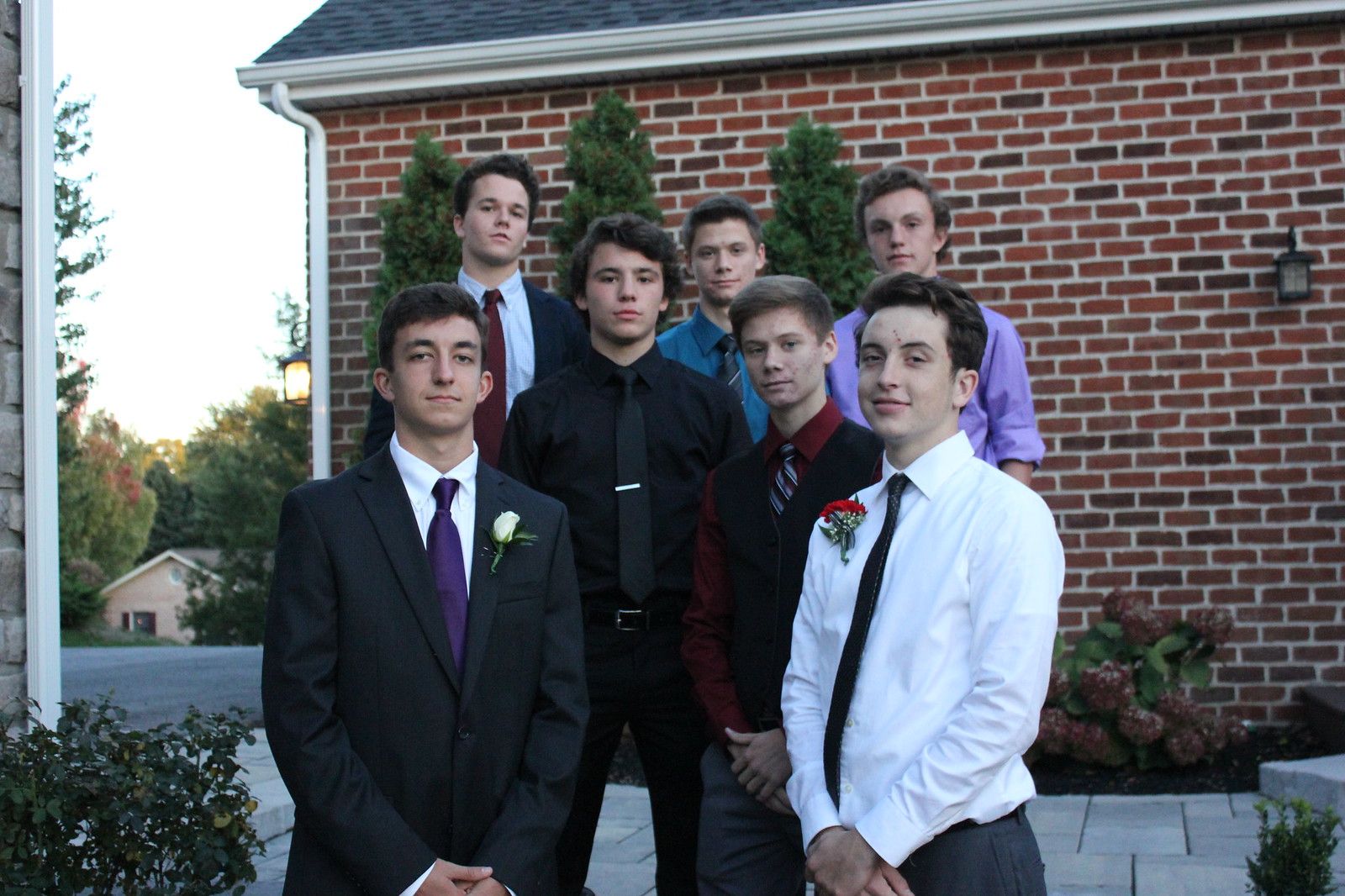This photorealistic image captures a group of seven young men, approximately 15 to 16 years old, dressed in formal attire, likely preparing for an event such as a dance or graduation. Centrally positioned, the group comprises individuals in suits, ties, and dress shirts of varied colors. In the front row stands a boy in a dark suit and purple tie, adorned with a boutonniere and sporting short brown hair. To the right, another boy wears a white shirt, black tie, and red flower boutonniere. Among the group, some boys wear only dress shirts and ties, with one notably in a burgundy shirt with a vest. The boys display somewhat forced smiles, suggestive of formal portrait etiquette.

Behind the boys stretches a red-brick house with a partially visible dark-colored roof. A small black lantern hangs on the exterior wall to the right. The setting features a silver interlocking stone walkway and a lush garden. On the right side, a large plant with green leaves and red flowers stands out, while further back three small green trees are planted. In the background to the left, a gray road, more green trees, and part of a small brown house can be seen, partially obscured by the foliage. The overall ambiance indicates an outdoor scene in the middle of the day.